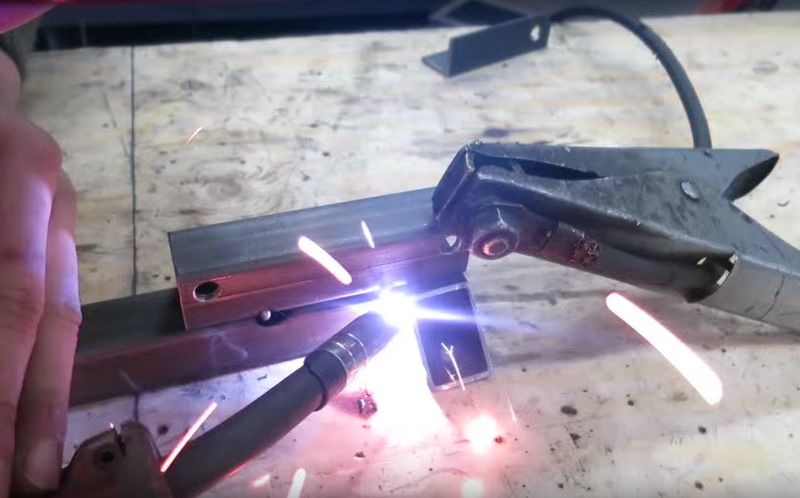In the image, a white Caucasian individual is holding an arc torch against a piece of metal, sparking bright white lines that emanate from the welding point. The individual is working on a white marble bench which provides a contrast to the dark grey metal clip secured with a bolt situated to the right. A black wire winds its way from the top right corner, crossing over and beneath the bench. Positioned at the top of the scene is a grey, square L-shaped metal piece, while a square metal piece with two holes is visible on the right side. Another square metal piece is located directly below it. A leg, likely bracing against the table, offers support. The arc torch, characterized by its silver front tip and black back end, emits an intense light at the junction of the two metal pieces, facilitating their fusion.